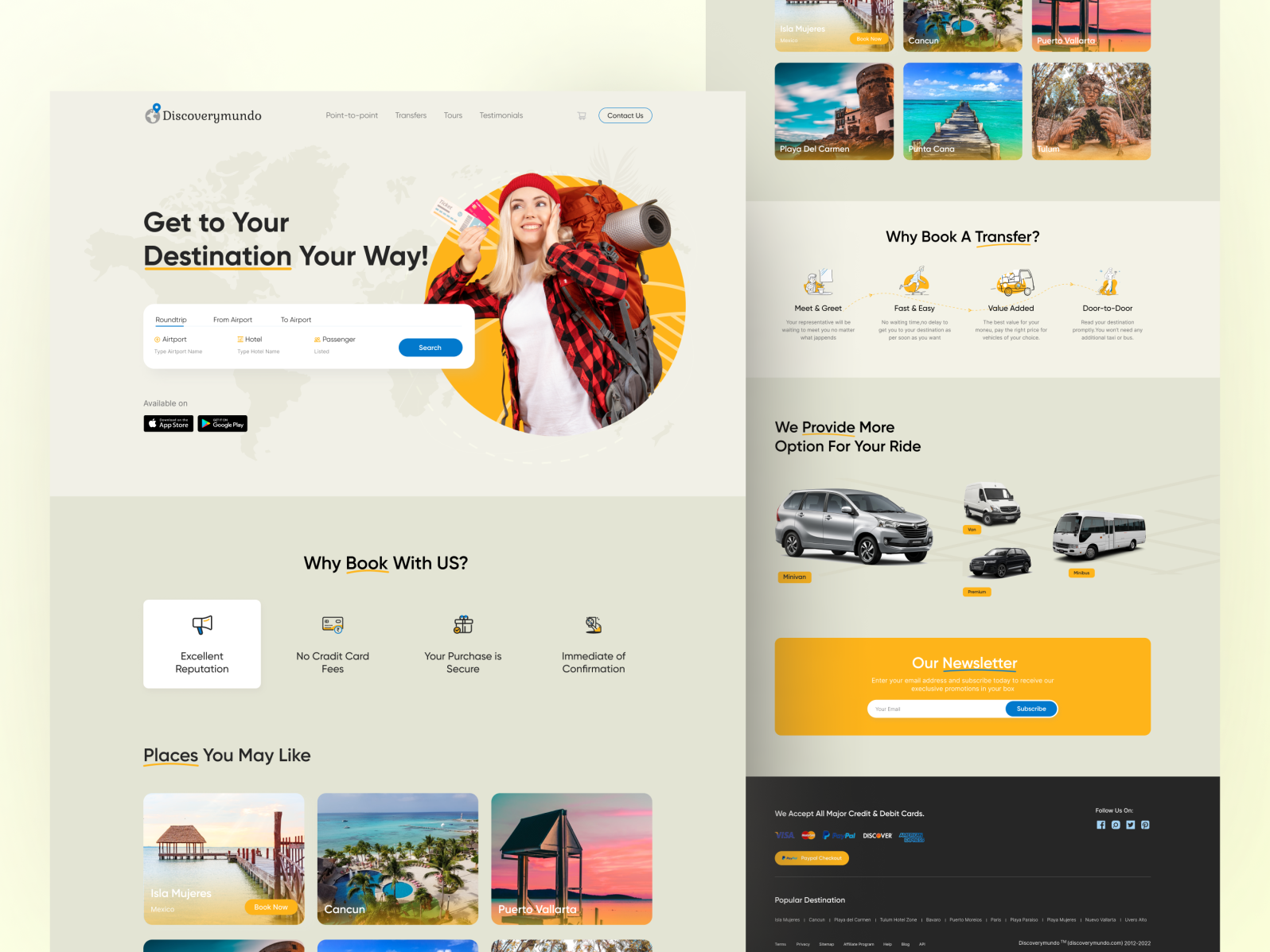Screenshot of the Discovery Mundo Website: The screenshot showcases a meticulously organized layout, resembling photo editing software where different pages are seamlessly blended together. The website is named 'Discovery Mundo'—a Spanish-tinged title, yet entirely in English. The main tagline reads "Get to your destination your way," with an interactive text field allowing users to input their desired destination, primarily targeting airport transfers.

Prominent links are visible for downloading Android and iOS apps. There are CTAs for purchasing services directly through the site, followed by an array of accolades such as "Excellent reputation" and "No credit card fees." The page is adorned with a mix of stock photos highlighting various destinations including Cancun and Puerto Vallarta.

Further sections of the site elaborate on the benefits of booking transfers, emphasizing speed, value-added services, and door-to-door convenience. The site positions itself as an all-encompassing travel solution, potentially covering flight bookings, hotel stays, and car rentals. The overall design features a modern layout set against a grayish background, giving it a sleek and professional appearance.